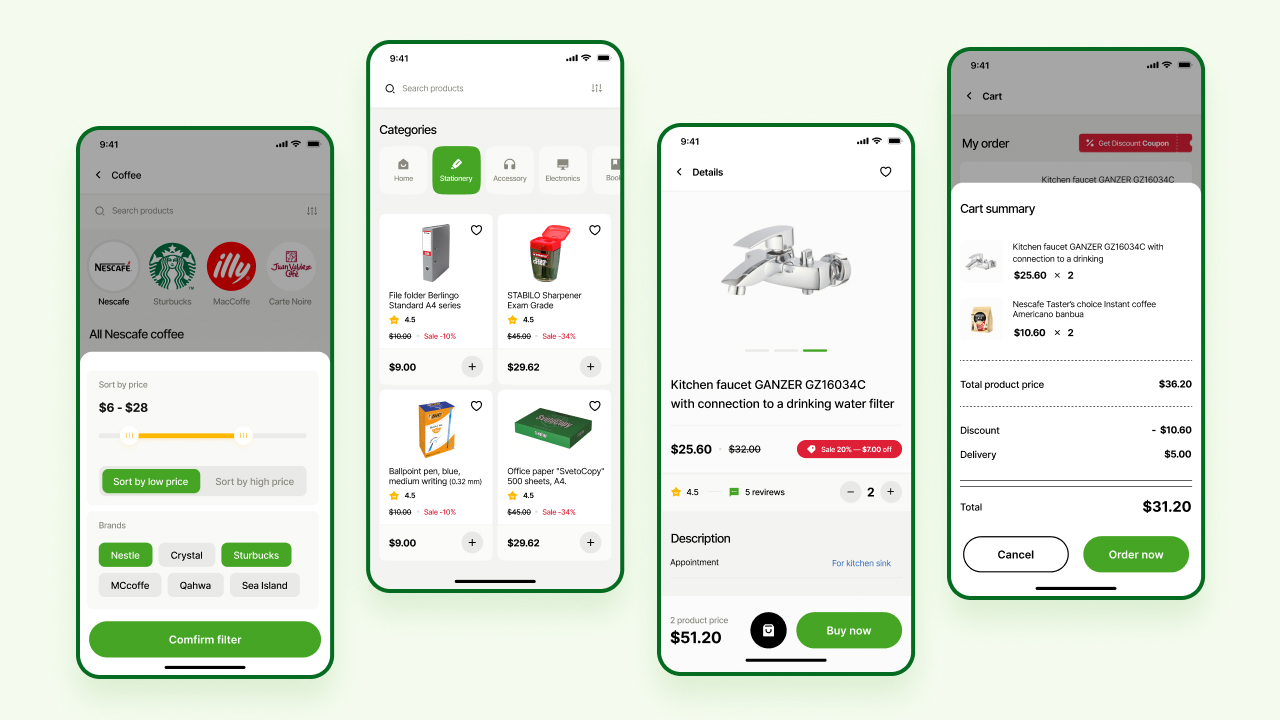Here's a polished and detailed descriptive caption for the image:

---

Against a light green backdrop, the image is a composite of four screenshots, presumably from a mobile application interface.

**Screenshot One:**
- **Background:** Off-white with a grayish hue.
- **Top Section:** A white pop-up bar with black text displaying a currency symbol, followed by "6-28".
- **Middle Section:** A half-filled yellow progress bar centered on the page.
- **Options Section:** Multiple blurred text options. The first row consists of a green bar on the left and a gray bar on the right.
- **Bottom Section:** Several controls, including a sequence of three options: a green box, a gray bar, and another green bar. Below these are three gray bars followed by a larger green bar displaying "Confirm Filter" in white text.

**Screenshot Two:**
- **Top Left Corner:** The word "Categories."
- **Tabs Section:** Five clickable tabs with the second tab highlighted in green.
- **Image Grid:** Two rows, each with two images:
  - **Top Left:** A tall, thin monitor.
  - **Top Right:** A black cup with a red lid.
  - **Bottom Left:** A yellow rectangular shape with a blue top.
  - **Bottom Right:** A green box.

**Screenshot Three:**
- **Product Highlight:** Silver faucet labeled with "Kitchen Faucet Ganzer GC76034C" in black text, followed by "with connection to a drinking water filter" and priced at $25.60.
- **Description Section:** Features a price tag of "$51.20" followed by a black circle. Additionally, there's a green bar with white text beside it.

**Screenshot Four:**
- **Cart Summary Section:**
  - **Contents:** An image of the previously mentioned silver faucet, priced at $25.90.
  - **Beneath the Faucet:** A gray bag associated with the list items, blurred and not clearly legible.
  - **Pricing Breakdown:** 
    - **Total Product Price**
    - **Discount**
    - **Delivery**
  - **Final Total:** "$31.20" in black text next to the label "Total."
  - **Actions:** A white bar with "Cancel" in black next to a green bar with "Order Now" in white.

---

This caption thoroughly describes each section of the image to provide a clear understanding of its content.